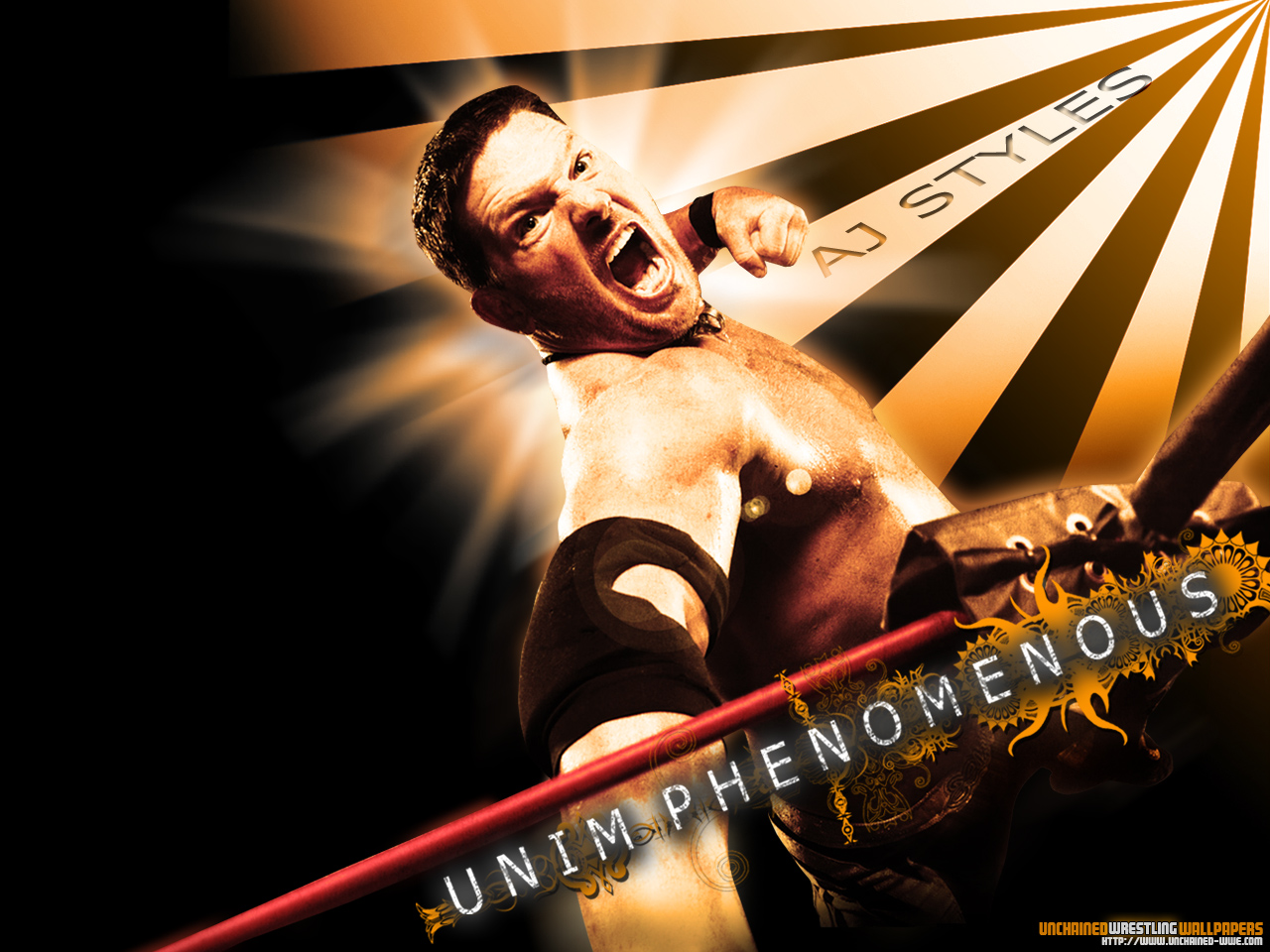The image appears to be a stylized, possibly edited, photograph intended for a computer wallpaper or advertisement. Central to the image is a dynamic photograph of the wrestler AJ Styles, captured from a low angle. He is depicted in mid-leap, with one arm stretched towards the viewer and the other cocked back, ready to deliver a punch, all while his mouth is open as if letting out a battle cry.

The composition features a striking gradient background that transitions from gold or orangish hues in the upper right corner to black towards the edges, giving the effect of sunlight filtering through. White and black lines radiate from the upper right corner, adding to the dramatic flair.

Text elements are prominently displayed: "UNCHAINED" is written in gold letters in the bottom right corner, followed by "Wrestling" in white, and "Wallpapers" in orange. Additionally, "AJ Styles" is inscribed in gray letters along one of the white lines descending from the upper right corner. Below the leaping AJ Styles, white letters spell out, "You and I am Phenomenal," with a red rope resembling a wrestling ring's rope positioned above the text. AJ Styles is also distinguished by wearing a black elbow pad, contributing to the wrestling theme of the imagery.